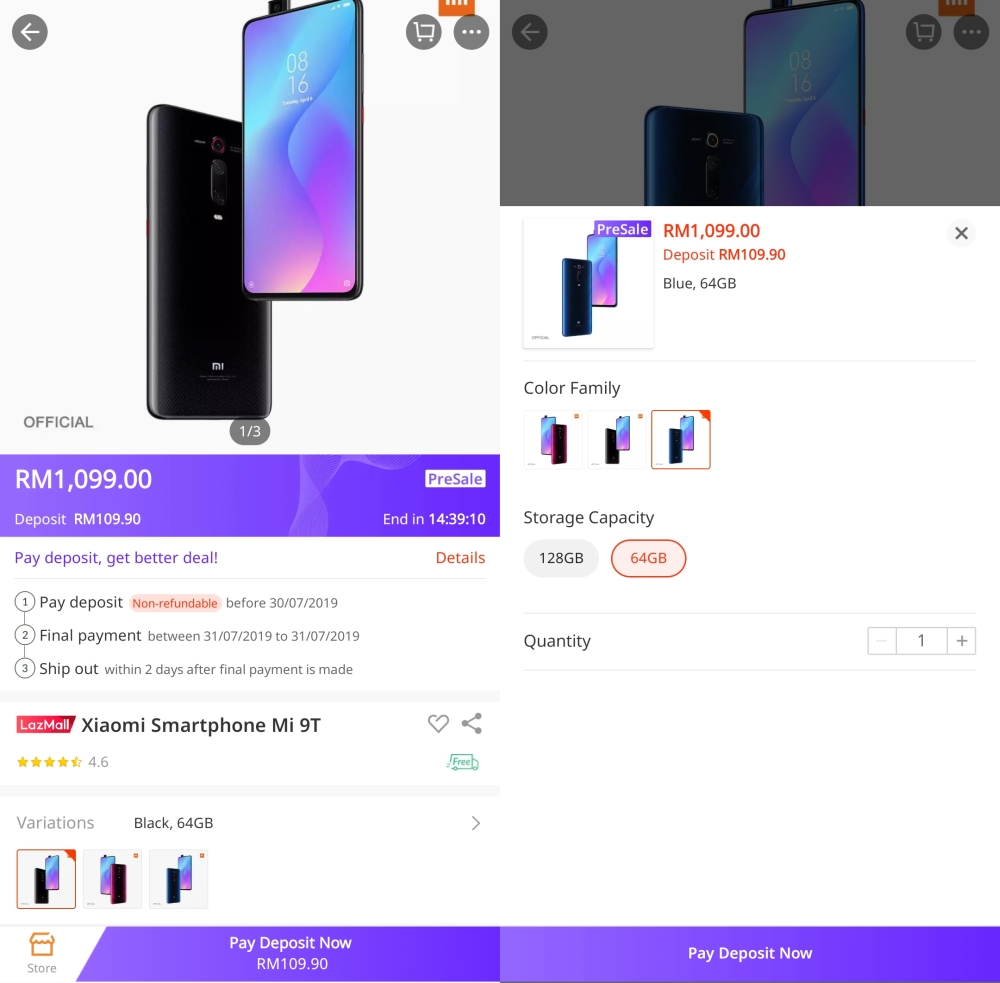Image Description: The image appears to be a screenshot from an e-commerce website, possibly Timu or another international platform, showcasing a Xiaomi smartphone available for pre-sale. 

Detailed Caption:
The image features a black Xiaomi MI9T smartphone, displayed with both front and back views. The phone screen shows a vibrant purple and blue gradient background with the time set to 8:16. The reverse side of the phone is sleek black.

Key promotional details are highlighted in a purple banner near the bottom of the image, indicating the phone is priced at RM 1099.00. The banner also mentions a pre-sale offer requiring a non-refundable deposit of RM 109.9, with the pre-sale ending in 14 hours, 39 minutes, and 10 seconds. The text elaborates that paying the deposit can secure a better deal.

Additional information outlines deposit terms: it must be paid before July 30, 2019, with the final payment due on July 31, 2019. The phone will ship within two days after the final payment is made. The product is sold through LAZ Mall and boasts a 4.6 out of 5 star rating, denoted by yellow stars. Shipping is free.

The image also details storage options, showing 64 GB and 128 GB variations, with the 64 GB option highlighted in orange. The bottom section features another purple banner prompting users to pay the deposit of RM 109.90 now to secure the pre-sale offer.

The combined elements suggest this is an auction-style or limited-time pre-sale event aimed at enticing early buyers with better deals and specific terms for purchase and delivery.